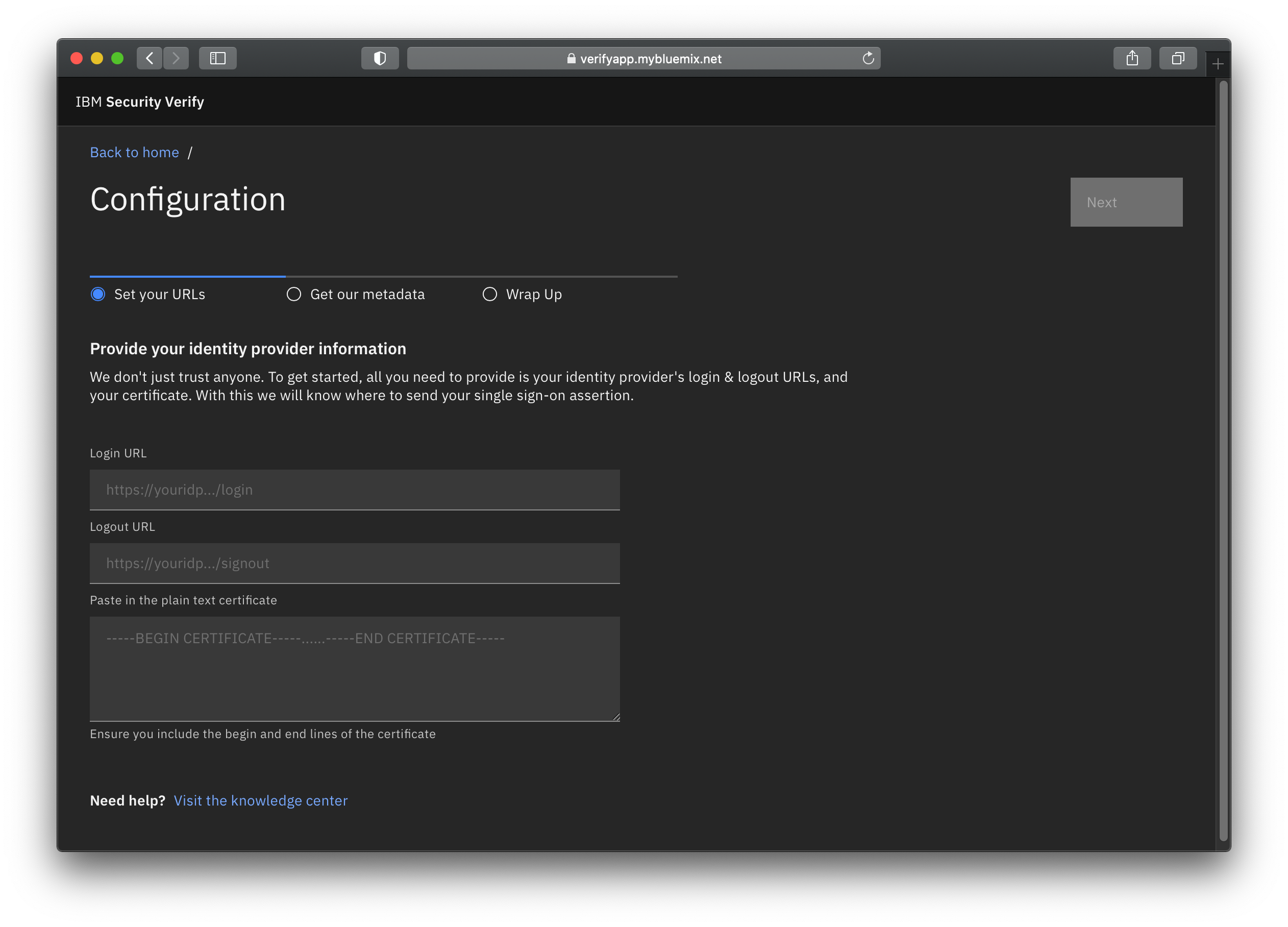The image displays an IBM Security Verify configuration page, accessed on an Apple MacBook, as indicated by the red, yellow, and green control buttons typical of the macOS interface. At the top of the page, the header reads "IBM Security Verify Configuration" against a subtle background. Below this, there is a search bar showing the URL `verify.bluemix.net`.

Prominently displayed on the page is a section labeled "Configuration" in large white text, which outlines a three-step setup process. Currently, the page is on "Step 1 of 3: Set Your URLs." The subsequent steps, "Get Your Metadata" and "Wrap Up," are listed below but not yet active. To the right of the "Configuration" heading is a grayed-out "Next" button, hinting that this step must be completed before proceeding.

The primary content area explains "Provide your identity provider information" in white text. It guides the user to input their identity provider’s login and logout URLs and certificate. Below this instruction, there are fields to enter the Login URL and a box to paste the certificate details, emphasizing that the beginning and end lines of the certificate must be included.

At the bottom left corner, there is a "Need Help?" section highlighted in bold white text, directing users to visit the Knowledge Center for further assistance. The "Knowledge Center" link is in blue, making it easily noticeable for anyone needing additional guidance.